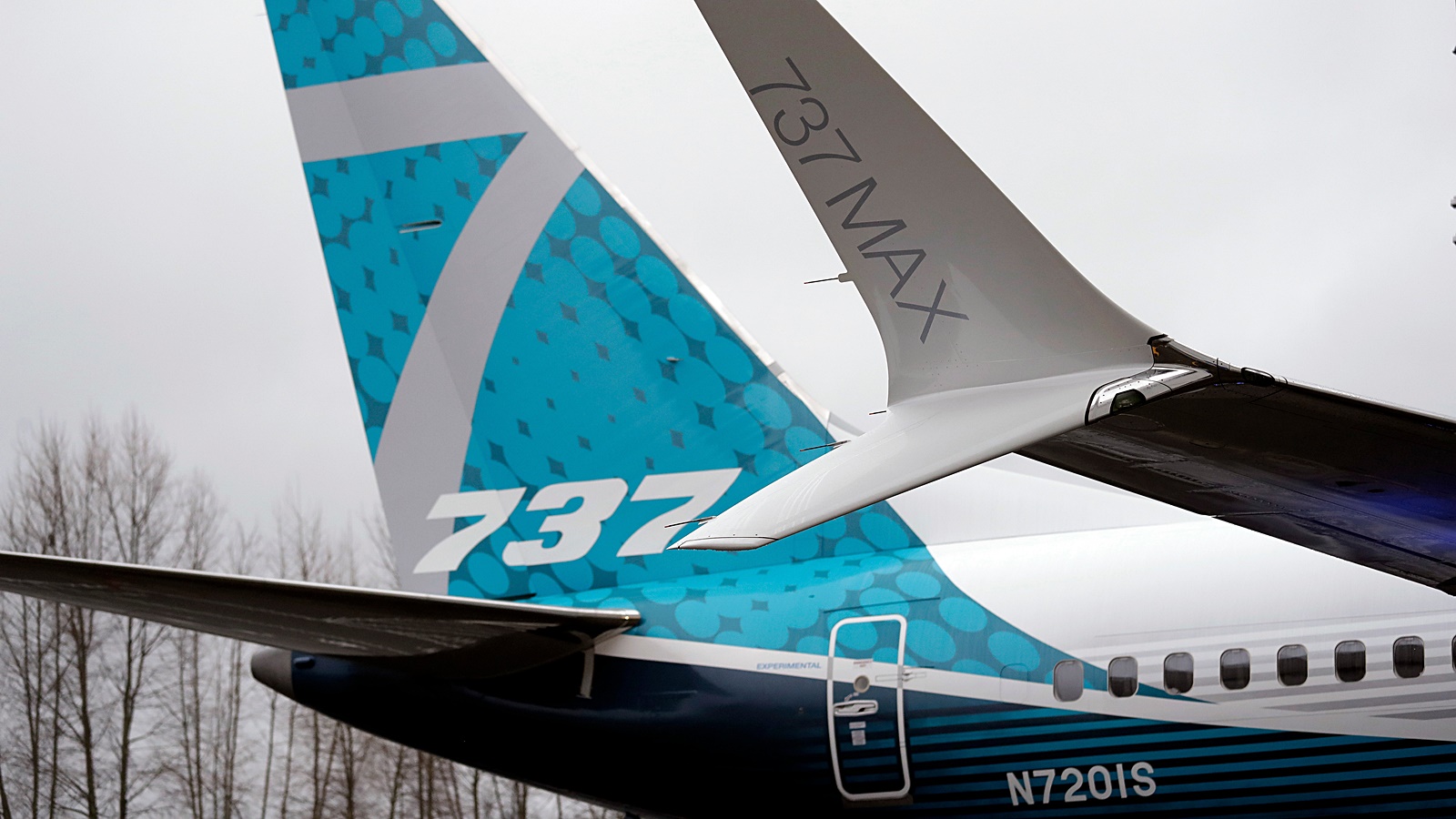The image captures the tail sections of two airplanes positioned outdoors against a featureless gray sky. The tail on the left belongs to a larger aircraft and prominently displays "737" along with the identifier "N7201S" beneath the windows. Adjacent to the door on this plane, another number "737 MAX" is visible. To the right, the smaller tail fin of a second aircraft can be seen, marked with "737 MAX" and featuring a blue, white, and black color scheme. In the background, the scene is bordered by a cluster of trees devoid of leaves, providing a natural contrast to the industrial setting of the planes. The perspective suggests the photograph was taken from a lower angle, emphasizing the grandeur and details of these aircraft tails.